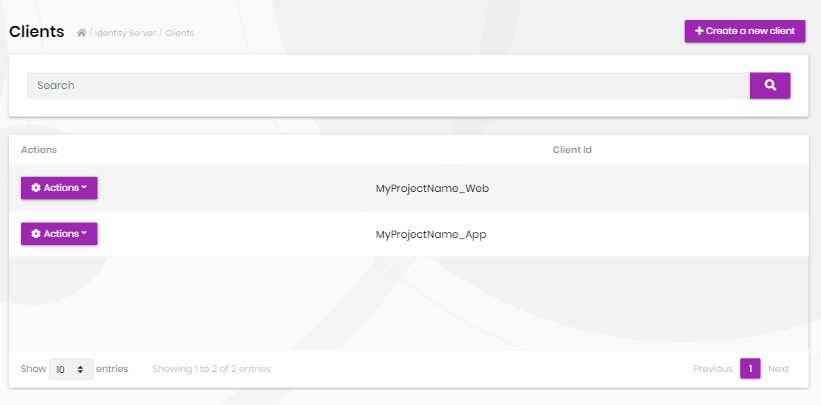The image depicts a webpage layout designed for client management. In the top left corner, the word "Clients" is displayed prominently in bold black letters. On the top right corner, there is a purple banner with the text "Create a New Client" accompanied by a white plus sign, indicating a clickable option to add new clients.

Below this header, there is a wide search bar with the placeholder text "Search". Adjacent to the search bar on the right, there is a small purple tab featuring a magnifying glass icon, denoting the clickable search function.

Beneath the search bar, a sizable white content box spans across the page. In the upper left corner of this box, the word "Actions" is visible. Within this box, there are two purple banners, each labeled "Actions". Both banners have dropdown arrows indicating clickable options. The first purple "Actions" banner is aligned with the text "my_project_name_web" in the middle section of the box. Similarly, the second purple "Actions" banner is aligned with the text "my_project_name_app" in the same middle section.